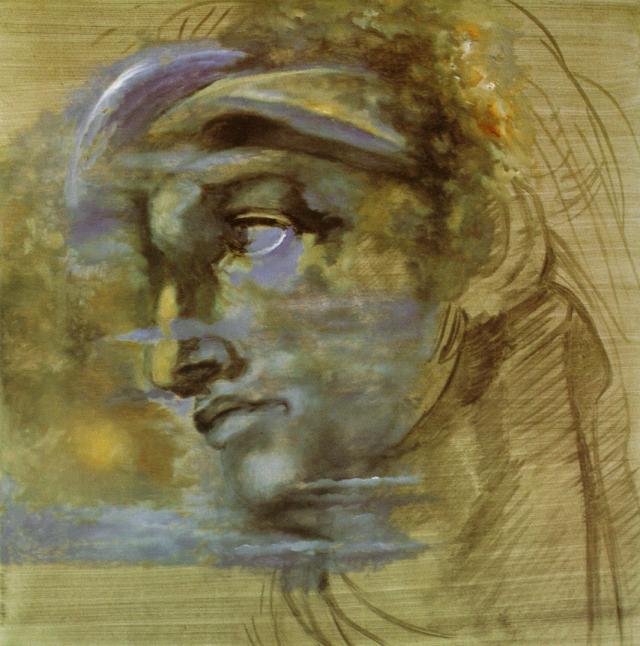This square piece of artwork, likely a drawing or painting, features a central image of a face that appears to be sculpted from stone, reminiscent of a Greek god or goddess. The face is depicted in profile, looking to the left, with a mix of gray and white tones, accentuated by subtle brown hues. These browns are particularly noticeable at the hairline, blending into what appears to be hair on top of the head. The hair is detailed with golden, curly locks, and is interspersed with streaks of silver and purple that curve gracefully over the forehead and to the right side of the head, almost resembling feathers. The background of the artwork is composed of varying shades of light brown, with subtle horizontal lines giving it texture. Minimal lines outline the neck and upper body, emphasizing that the primary focus is the face. Additional colors dispersed throughout the image include white, tan, yellow, green, orange, red, and purple. The scene is devoid of any text, placing full emphasis on the striking, central face, evocative of classical statue.